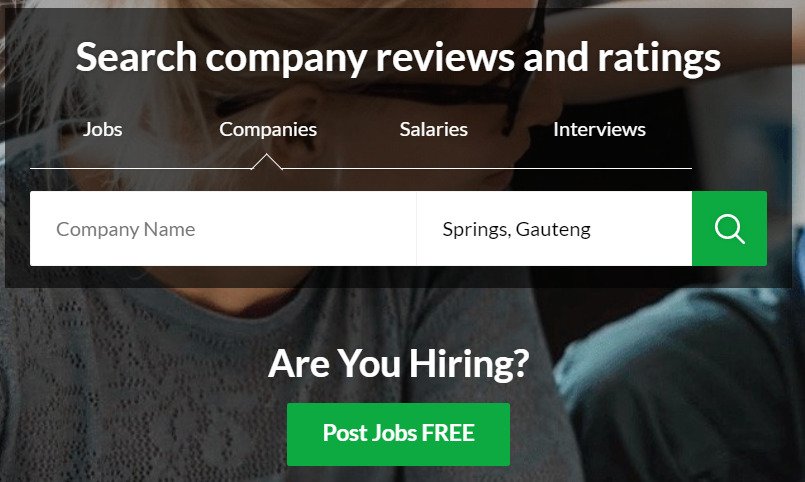The image, likely designed for a website or app, features a horizontal layout that is approximately 30% wider than it is tall. The background serves as a banner image, showcasing an elderly Caucasian woman. The woman's face and upper body are visible from the top of her chest to the middle of her forehead. Positioned on the left-hand side of the frame, her body faces the viewer but her head is turned to the left, gazing at the three o'clock direction. She has gray hair and is wearing black glasses along with a gray long-sleeved shirt. Her figure occupies roughly two-thirds of the image's width.

In the background, there is a glimpse of another person, identifiable only by their right shoulder clad in a teal shirt.

Overlaying the image is a semi-transparent gray box that extends down about two-thirds of the image from the top. At the very top, the text reads "Search company reviews and ratings." Below this are four menu options labeled "Jobs," "Company," "Salaries," and "Interviews." The "Company" option is highlighted with a small up arrow beneath it. Beneath these menu options, there is a search bar with the placeholder text "Company name" and to the right, "Springs, Gauteng."